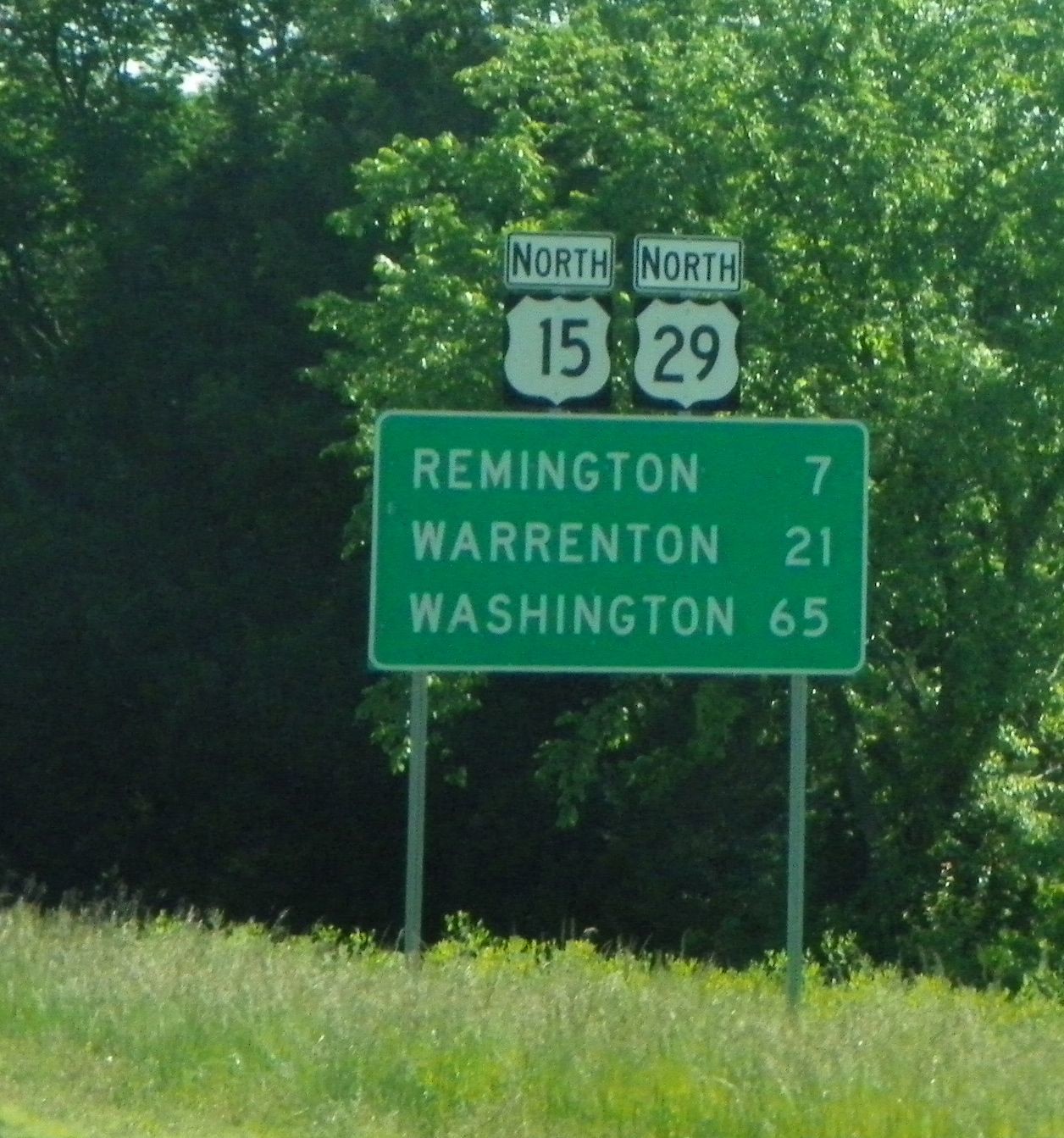The photograph captures an angled view of a road sign situated in a lush outdoor area, flanked by tall green grass and dense trees in the background. The foreground features abundant tall green grass and weeds, while the background consists of a verdant forest. The central focus of the image is a green rectangular directional sign with white text, mounted on two slender metal poles. The sign lists three cities and their respective distances: "Remington 7," "Warrington 21," and "Washington 65." Above the green sign are two smaller black and white highway symbols, indicating "North 15" and "North 29," positioned side by side. The scene is brightly illuminated by daylight, showcasing the vivid colors and details of the natural surroundings.